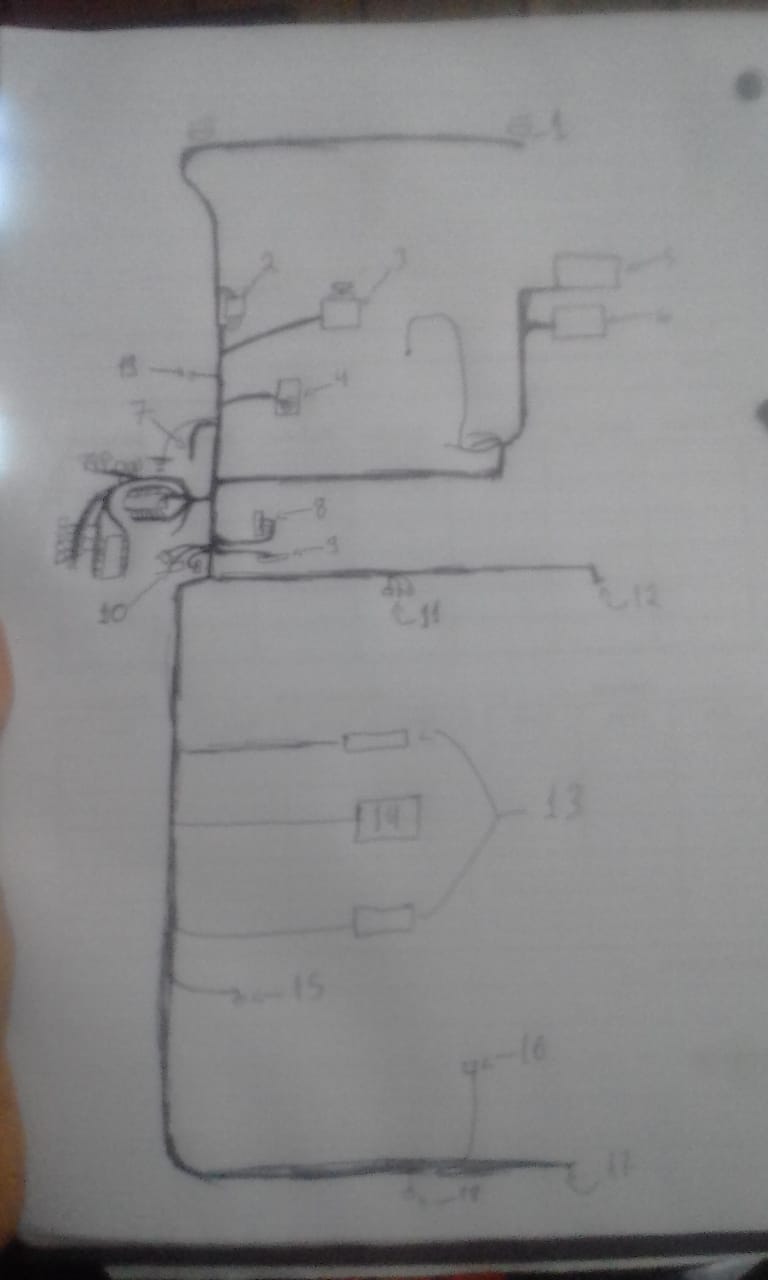A blurry photograph captures an exercise book lying open, featuring a page with perforated holes neatly removed from its right edge, designed to fit into a binder. The page showcases a pencil-drawn circuit diagram with the overall layout resembling a backward "E." The diagram is intricate, with thicker black lines branching into finer lines that either lead to small rectangular boxes or terminate in tiny dots scattered across the page. Each rectangle is annotated with numbers and arrows, providing specific details about the circuit elements. Some thicker lines are shorter and split into additional branches, which are adorned with small circles on sticks, evoking a bottle brush appearance. The complexity and detail of the diagram occupy the entire page of the exercise book.